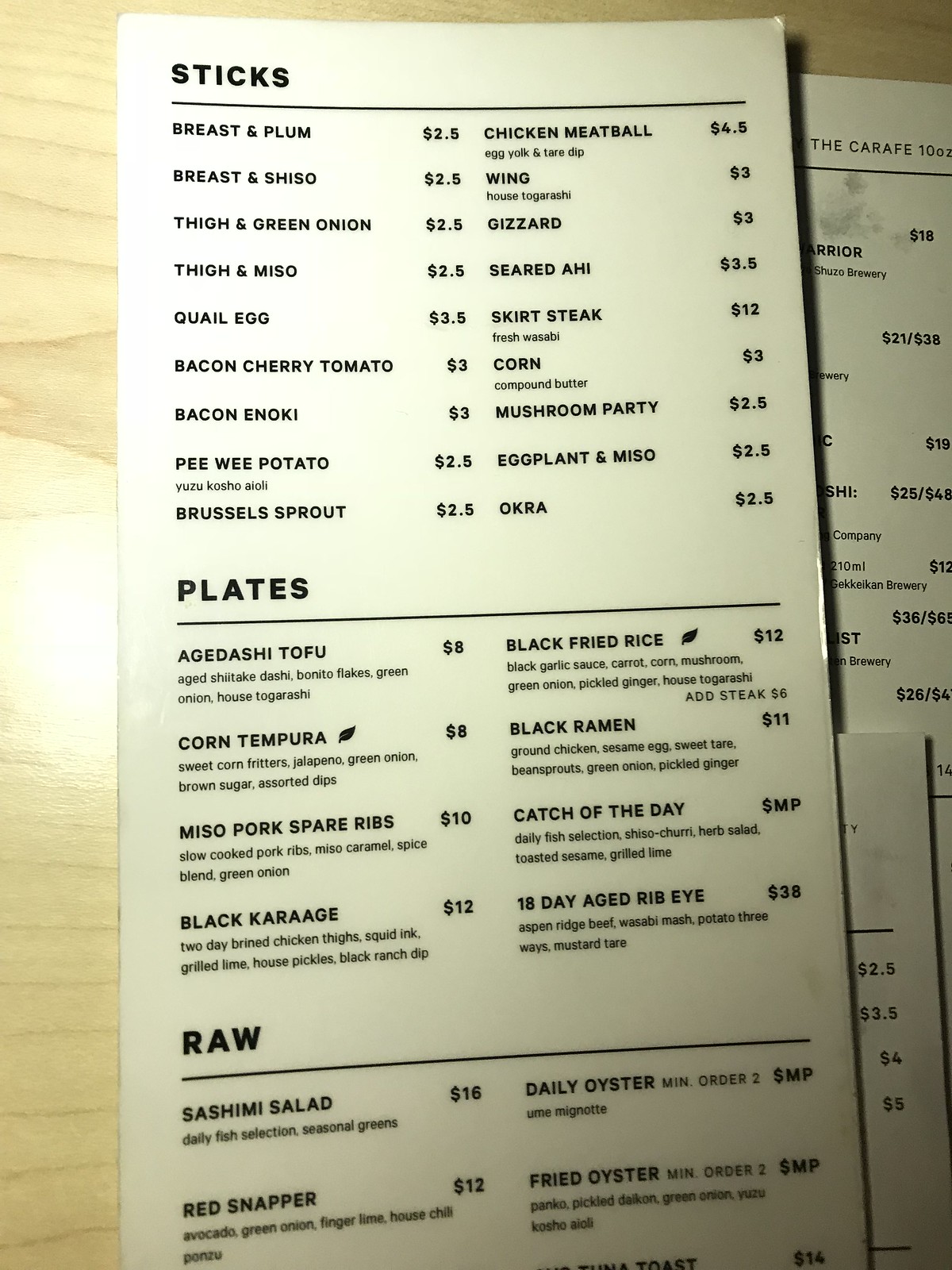The image captures a detailed photograph of a restaurant menu laid on a light wood-colored tabletop. The black-and-white menu features a variety of enticing dishes, divided into distinct categories. At the top, the "Sticks" section includes flavorful options such as Breast & Plum, Breast & Seashell, Thigh & Green Onion, Thigh & Miso, Quail Egg, Bacon-wrapped Cherry Tomato, Bacon-wrapped Enoki, Peewee Potato, and Brussel Sprouts. 

Below, the "Plates" section offers enticing dishes like Agedashi Tofu, Corn Tempura, Miso, Pork Spare Ribs, and Black Karaage. Further down, the "Raw" section lists fresh seafood selections including Sashimi Salad, Red Snapper, Daily Oyster, and Fried Oyster. 

The menu appears to be resting on additional menus or possibly other pages of the same menu, hinting at a broader array of dishes not fully visible in this specific snapshot. The overall setting suggests a casual dining experience with a focus on varied and appetizing selections.